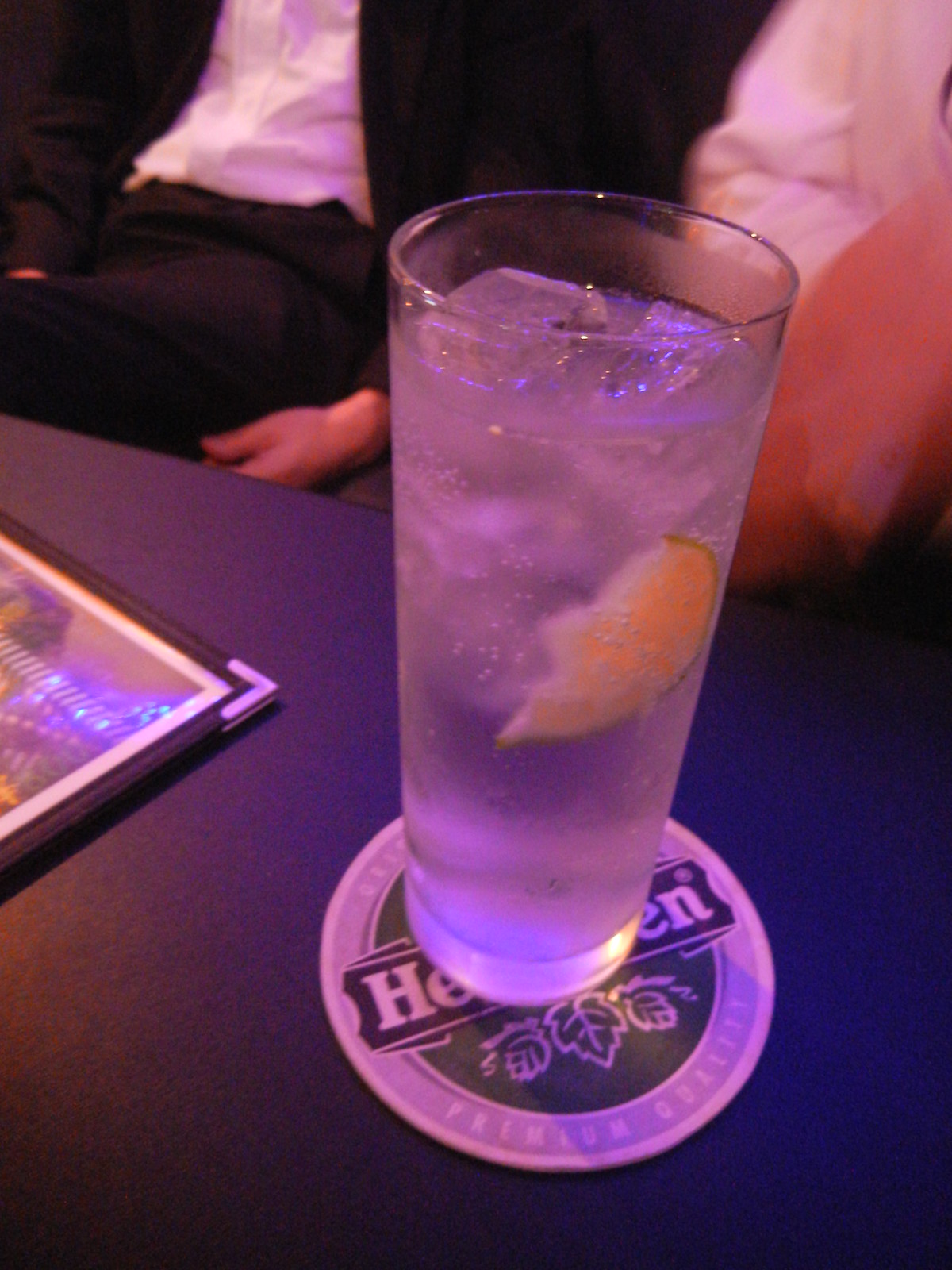This detailed color photograph, shot in portrait orientation, prominently features a tall glass of clear ice water with a lemon slice, placed on a circular Heineken coaster atop a black table. The Heineken coaster is distinguishable with its dark green background, white border marked with gray stripes, and the brand's logo in black across the center. Next to the glass, a segment of a restaurant menu is visible, notable for its protective metal corner. The photograph captures two seated individuals, focusing only on their mid-sections; both appear to be male, with one in a black suit paired with a white shirt and the other visible only by his arm clad in a white shirt. The setting suggests an indoor venue, likely dimly lit, such as a bar or restaurant.